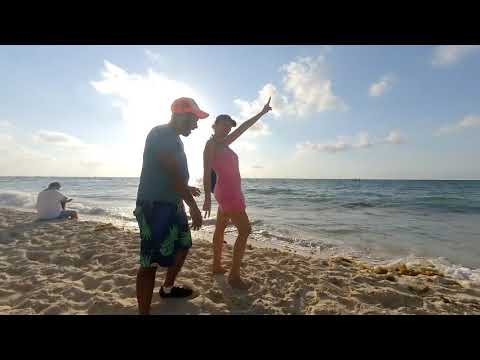This outdoor daytime photograph features a vibrant beach scene framed with black stripes along the top and bottom, giving it a panoramic effect. In the foreground, three individuals are captured on the well-trodden sandy shore. Central to the image is a woman with lighter skin, dressed in a pink sundress and a black ball cap. She strikes a playful pose, pointing her left index finger skyward while her right hand makes a V-shape towards the ground. To her left stands a man with darker skin, partially obscured by lighting. He is adorned in a short-sleeve gray or blue shirt, a red or orange ball cap, and distinctive blue swim trunks patterned with green pineapples. He wears black shoes and appears to be leaning towards the woman, looking down. To the far left, at the intersection of the sand and the incoming tide, sits another figure. Seen from behind, this person sports a short-sleeve white shirt and dips their feet into the gentle waves. The background showcases the serene ocean meeting the sky, which is painted with clouds radiating outward from the center, suggesting a bright, sunny day with a few clouds dotting the blue expanse. The scene is vividly detailed, capturing the essence of a lively, sunny day at the beach with its unique characters and dynamic poses.